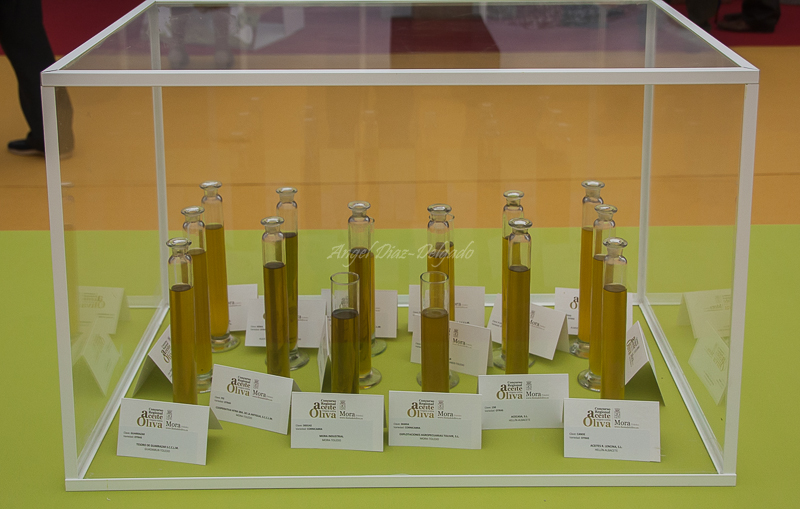The photograph showcases a rectangular clear display case, made of glass or perspex with aluminum corners, creating a three-dimensional effect. The case is open at the bottom and is placed on a greenish-yellow tablecloth that visually splits the image horizontally, with an orange-toned floor reminiscent of a school gym visible beneath. Inside the case are 14 tall, narrow vials, resembling test tubes, most with white and silver caps, although two remain uncapped. These vials appear to contain a liquid, possibly oil or perfume. Strewn around the vials are business cards or envelopes, mostly unreadable, listing names like Oliver and Mora. In the background, a pair of legs clad in brown pants and black shoes stand visible from the thigh down, adding a human element to the scene. Additionally, a dark maroon band at the very top of the image suggests a wall or partition, providing depth to the setting.